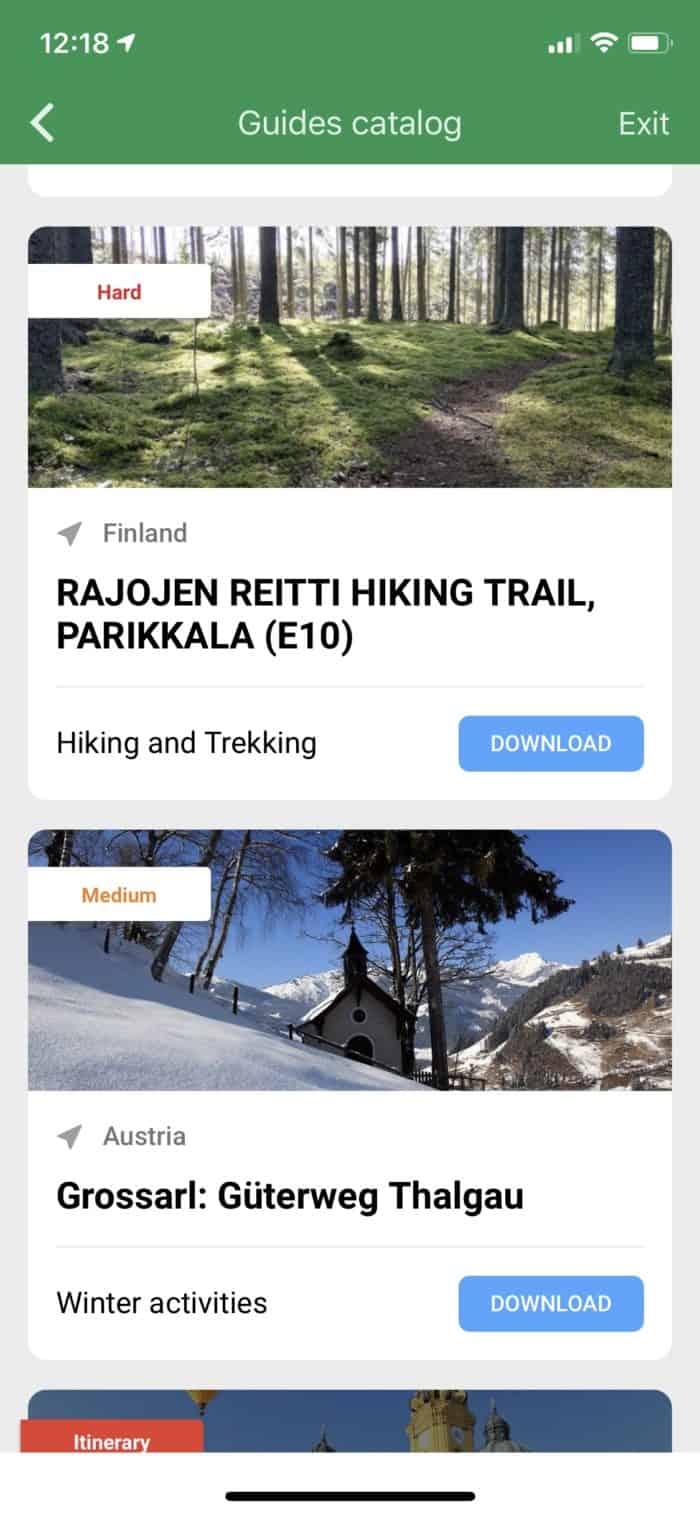The screenshot displays a mobile application's interface under the section labeled "Guides Catalog". The status bar at the top of the screen has a green hue and indicates the time is 12:18, with the battery life showing approximately 75-80%. 

The first entry features an image of a woodland path bathed in sunlight filtering through dense trees. This entry is labeled as "Hard" with the title "Rejogen Rieti Hiking Trail, Peräkäla". The trail is categorized as E10, located in Finland, and is suggested for hiking and trekking. 

Below the first entry, there is another listing classified as "Medium". It showcases a picturesque snowy scene of a quaint church in Austria, titled "Grossar Gutterweg, Falgau". This entry highlights winter activities available in the region, potentially for exercising. 

A blue download button is visible but partially cut off, indicating there are more entries to explore upon scrolling. The section is described as "Itinerary", suggesting these are various routes, activities, and destinations available for users, although specific details about the opportunities or interactions with locals are not mentioned.